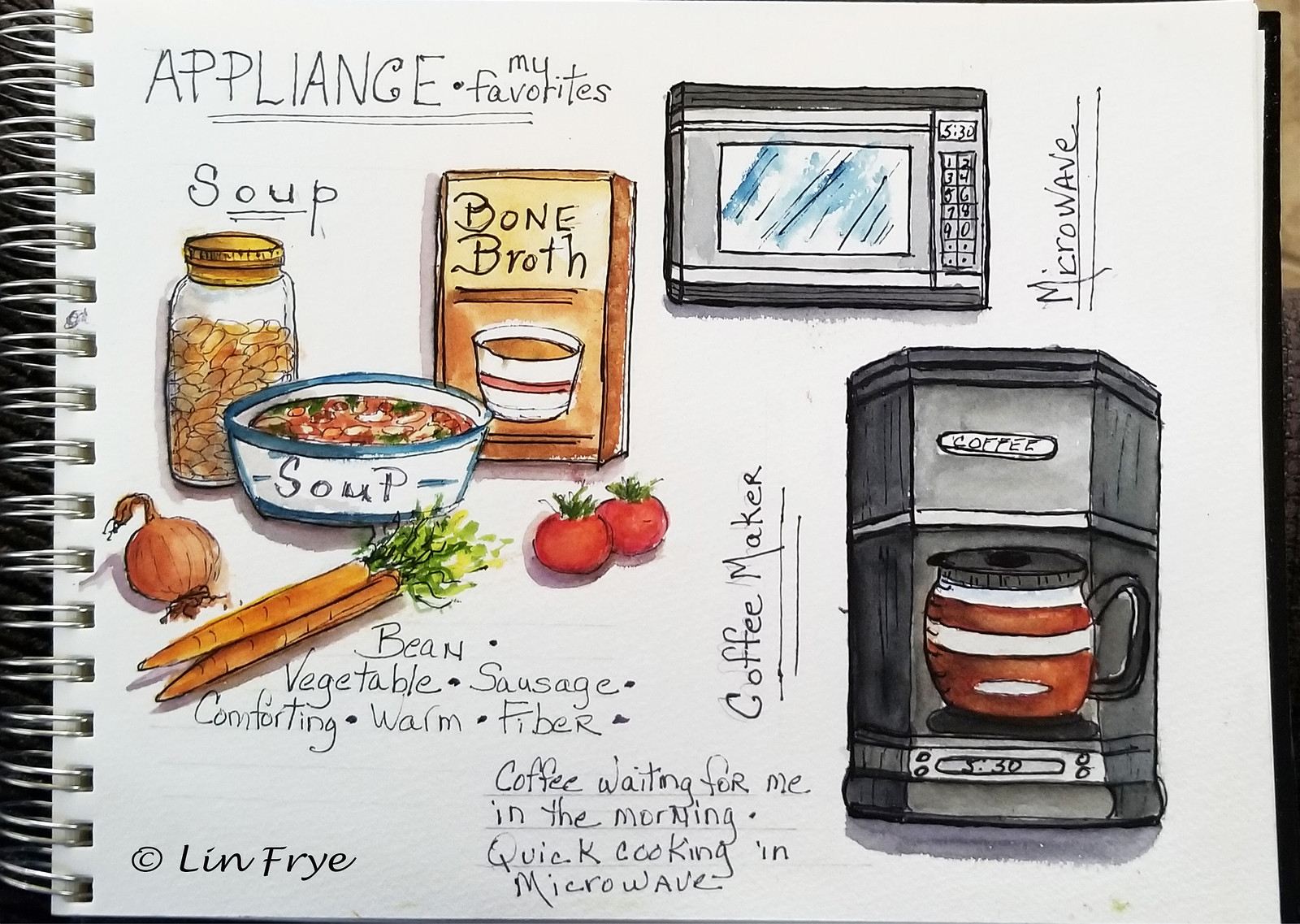An intricate illustration is captured on the pages of a notebook bound with multiple rings on the left side. The top left corner features a section labeled "Appliance by Favorites." Adjacent to this, on the top right, is a depiction of a microwave. The microwave is shown from a side view with white lines on top, contrasting against a black body, along with a glass window. A clock display is visible on the right side of the microwave.

Below the microwave, in the bottom right corner, there is a depiction of a coffee maker. The coffee maker features a brown pot and is labeled with the word "coffee." It is a large machine with a three-sided display at the bottom reading "3:30" with dots flanking the numbers, and a silver middle section.

Descriptions are noted in the bottom left, such as "coffee waiting for me in the morning" and "quick cooking in the microwave." Illustrated to the upper left is a jar labeled "bone broth," indicative of soup, with a white cup containing a brown liquid beside it. Further left, another soup illustration appears, described as a "white soup," accompanied by its various components.

The ingredients are visually detailed at the bottom left: an onion, a green carrot with leafy greens, an orange carrot with green leaves, and a red tomato with greens on top. Descriptive words like "bean," "vegetable," "sausage," "comforting," "warm," and "fiber" are scattered around, capturing the essence of the illustrated contents.